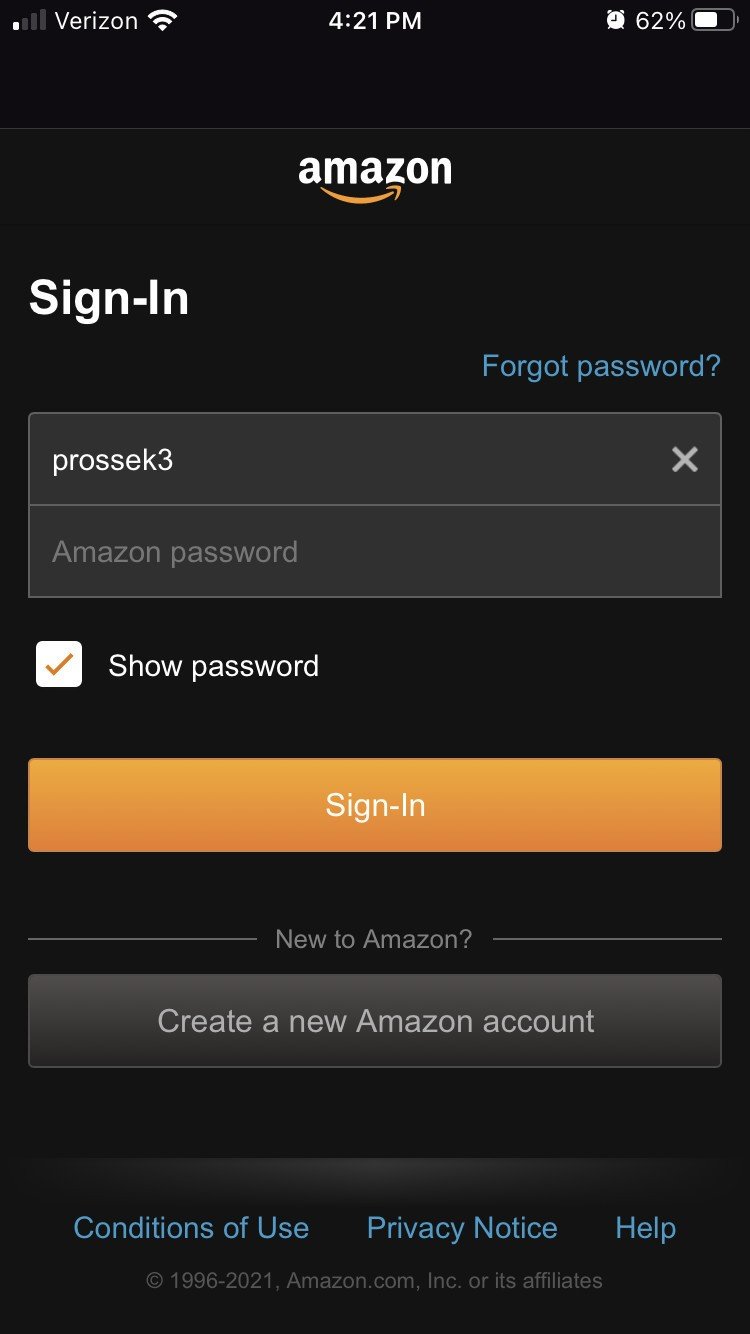This is a detailed description of a screenshot from the Amazon sign-in page on a smartphone. 

The interface displays a single sign-in form with two text fields for the username and password. The username field contains the text "prosec3", while the password field has a placeholder text indicating where the user should enter their Amazon password. Positioned below the password field is a checkbox labeled "Show password," which is checked. Directly below this checkbox is an orange button labeled "Sign-In," and further down, a gray button for creating a new Amazon account.

To the right of the password field, there is a link labeled "Forgot my password." Below the Sign-In button are three additional links: "Conditions of Use," "Privacy Notice," and "Help." 

The page's footer reads "1996 to 2021 Amazon.com Inc. or its affiliates." At the top of the page is the Amazon logo, with the heading "Sign-In" centered beneath it. The username and password fields are centered below this heading. The entire background of the interface is black, in keeping with Amazon's typical mobile app design, which emphasizes a clean and minimalistic style. The primary colors used are gray and orange, and all text on the screen is clear, legible, and presented in a consistent font.